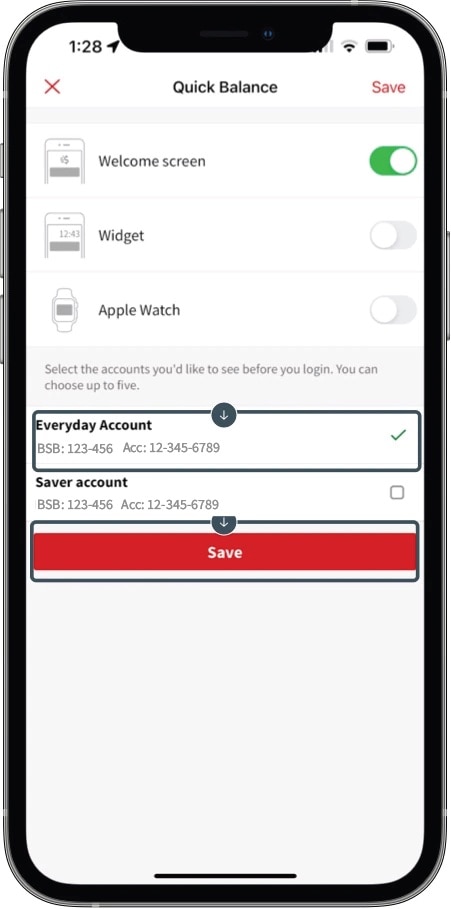This is a detailed screenshot of someone's smartphone interface. The image captures the entire phone with a distinct black outline around its edge. The phone's screen is predominantly white, featuring black text and various icons. 

In the upper-left corner, the time is displayed as 1:28, accompanied by a small black direction arrow. On the upper-right side, there are icons for the internet connection and battery status. Centered near the top, the text "Quick Balance" appears in black, flanked by a red "X" on its left and a "Save" button on its right.

Below this header, the screen displays the label "Welcome Screen" alongside a phone symbol and a movable green dot. This is followed by the word "Widget," next to which appears a toggle switch for turning a feature on or off.

Further down, there is an "Apple Watch" section, illustrated by an Apple Watch icon on the left and another toggle switch to enable or disable the feature. Under these sections, additional text reads: "Select the accounts you'd like to see before you log in. You can choose up to five."

The user has selected the "Everyday Account," marked by a set of numbers underneath and a green checkmark on the right side. Below, the "Saver Account" is listed with an empty gray checkbox that can be clicked. At the bottom of the screen, there is a prominent red "Save" button, bordered by a thick black line, indicating that it has been pressed.

Overall, this screenshot illustrates the various settings and selections available to the user, emphasizing their choices and the available customizations for a quick balance view on their phone.